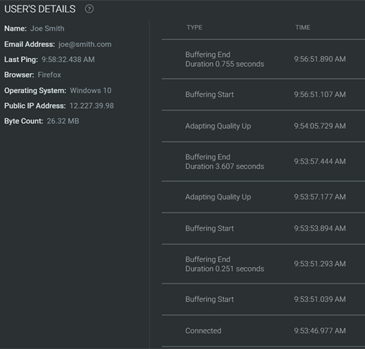Detailed Caption: 

The image is a screenshot of a user activity interface, presenting a black background adorned solely with text, primarily in white and grey hues. In the top left corner, the interface categorically displays the label "USERS DETAILS" in all caps, accompanied by a question mark encased in a circle, indicative of a help or information button.

Beneath this heading, a bordered section contains eight pieces of user-specific information listed vertically:

1. **Name:** Joe Smith
2. **Email Address:** joe.smith.com
3. **Last Ping:** 958.32.438 AM
4. **Browser:** Firefox
5. **Operating System:** Windows 10
6. **Public IP Address:** [number redacted]
7. **Byte Count:** 26.32 MB

Adjacent to this section are two additional vertical columns. The first column begins with:

- **Type:** Buffering Start
- **Time:** 9.56.51.890 AM

This pattern continues down the column, documenting various events and their corresponding timestamps:

1. **Buffering Start:** 9.56.51.890 AM
2. **Adapting Quality Up:** [Time]
3. **Buffering End:** [Time]
4. **Adapting Quality Up:** [Time]
5. **Buffering Start:** [Time]
6. **Buffering End:** Duration 0.251 seconds, [Time]
7. **Buffering Start:** [Time]

Each entry is separated by a grey vertical line, clearly segmenting the information. All timestamps indicated are in the AM period around 9:53-9:56. The detailed layout and chronological events suggest a tracking of user interaction over a given period, highlighting network activity, buffering states, and quality adjustments.